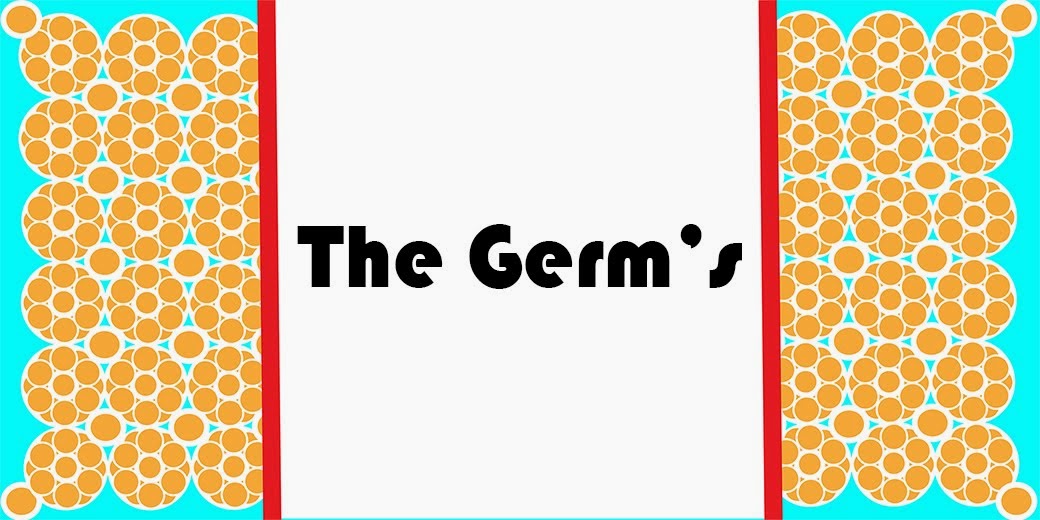This poster features a symmetrical design with a white central section flanked by patterned borders. The edges of the poster have an aqua-colored background adorned with repeated patterns of orange circles that resemble flowers, each consisting of a larger central circle surrounded by six smaller ones. These patterned columns are arranged three across and six down on either side. Bold red lines separate these intricate designs from the central white square. The middle white section of the poster prominently displays the title "The Germs" in bold black font, with both 'T' and 'G' capitalized. The design elements—including the orange circular patterns and red barriers—suggest a visual representation of germs and the barriers preventing them from spreading.